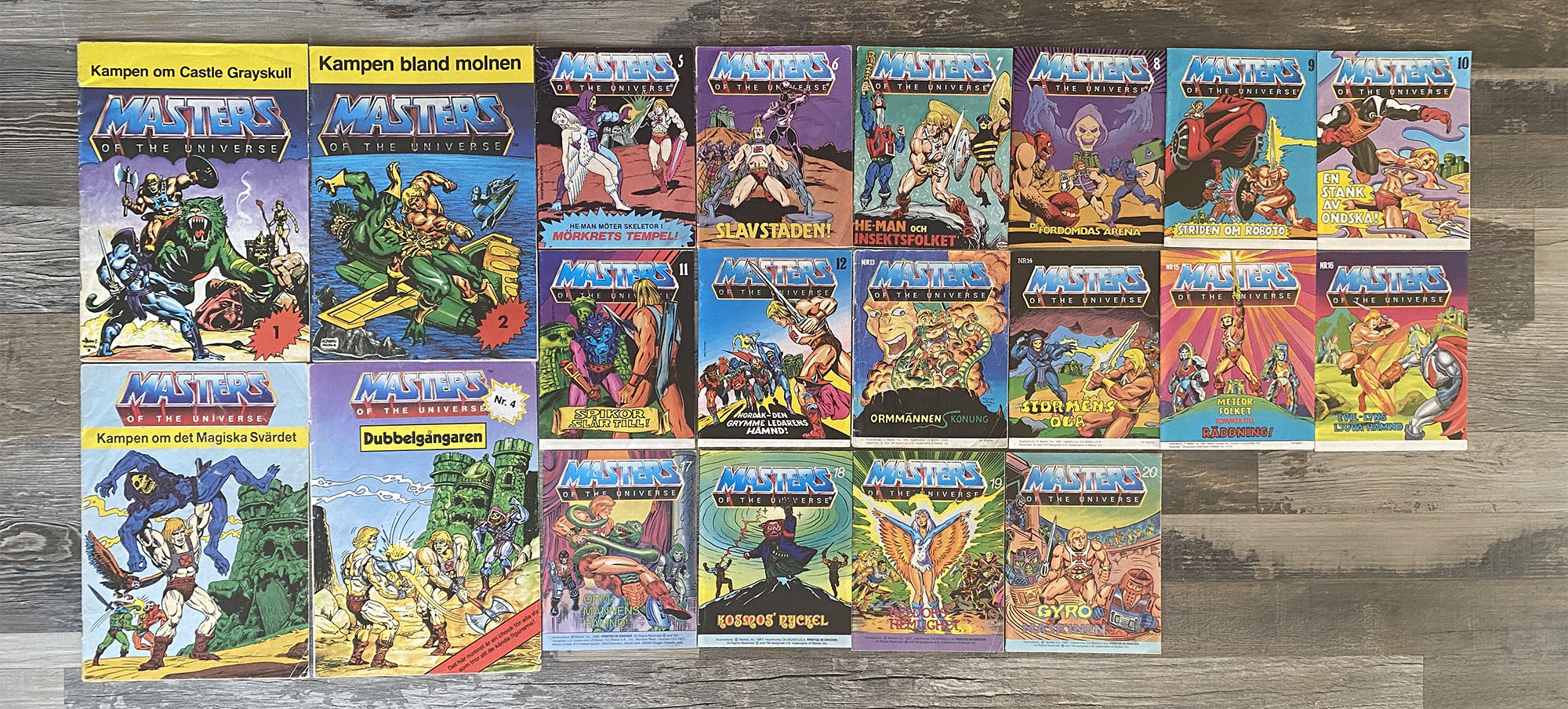This image features a bird's eye view of an assortment of comic books displayed on a brown, wooden, tile-like floor. Dominating the left side are four larger comic books, each branded with the title "Masters of the Universe" in bold blue letters at the top. These larger books feature different characters, including He-Man, often depicted in various dynamic poses—sometimes wielding a sword, sometimes simply using his fists. The book covers illustrate a range of creatures and scenarios, such as a green, bear-like animal clashing with a blue mythical beast. 

To the center and right are smaller comic books arranged in rows—six in the first, six in the second, and four in the third. Their covers showcase a vibrant palette of colors, including dark blue, purple, cyan, orange, red, green, and pink. They feature retro fonts and drawings, emphasizing a cartoonish and nostalgic aesthetic. One particularly striking cover features cascading stripes of red and orange with He-Man holding his sword aloft, capturing the essence of dramatic comic book action.